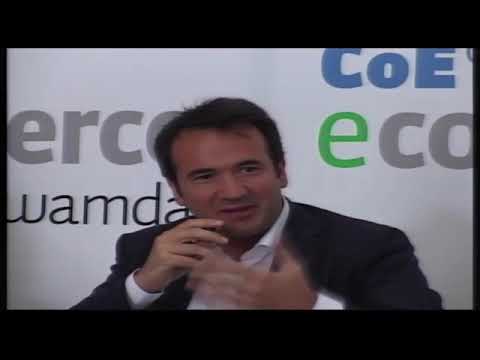This color photograph, resembling a screen capture from a video, features black widescreen bars at the top and bottom. In the center of the image, a man with tanned brown skin and slightly messy, short black hair sits in front of a white wall adorned with large, partially legible lettering, including "C-O-E" in blue, "E" in green, "C-O" in gray, "E-R-C" in green, and "W-A-M-D-A" in black bold text.

The man, appearing to be on a stage or at a conference, is wearing a dark gray or deep navy blue suit jacket with a white dress shirt underneath. A notable feature is the blue or purple handkerchief in his left breast pocket. He is holding a microphone near his mouth with his right hand, suggesting he is speaking or responding to questions, while looking slightly to his left, to the right side of the photograph. Additionally, a partial shadow of the man is visible on the wall behind him, and a microphone is attached to his collar, with its cord discernible.